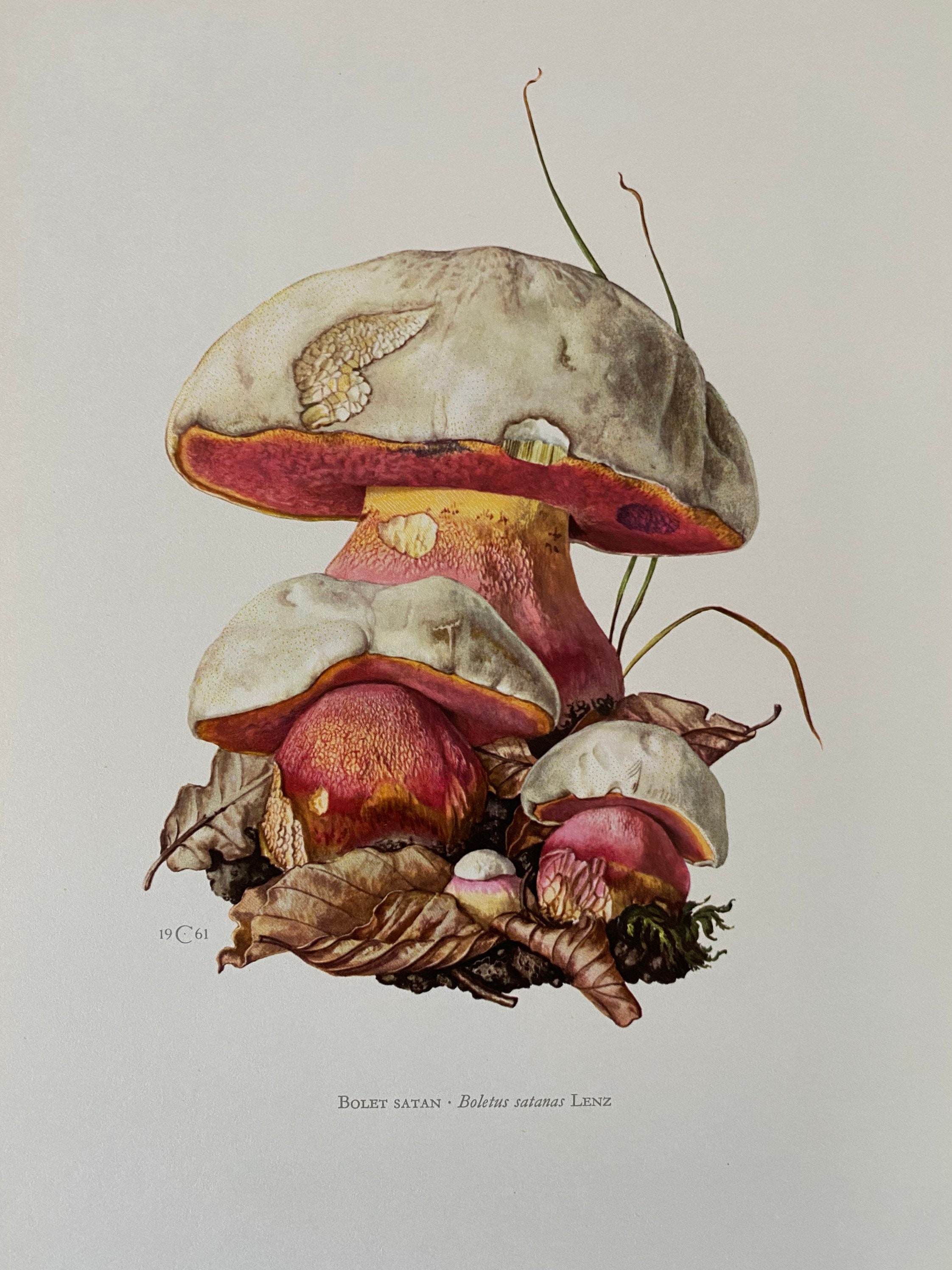This detailed illustration depicts a cluster of hand-drawn mushrooms set against a white background. The focal point is a large, central mushroom with an off-white, slightly browned cap featuring numerous indentations. The underside of the cap is vibrant red, encircled with a yellow-orange ring, while the stalk displays a gradient of red, pink, and yellow hues. Adjacent to it are two progressively smaller mushrooms, similarly colored with off-white, browning caps and red-tinted stems. These mushrooms are nestled atop withered, brown autumn leaves and scattered blades of grass, adding to the naturalistic setting. The artwork, evocative of a toadstool and titled "Boletus Satanae," includes the name boldly across the bottom, enhancing its botanical accuracy.